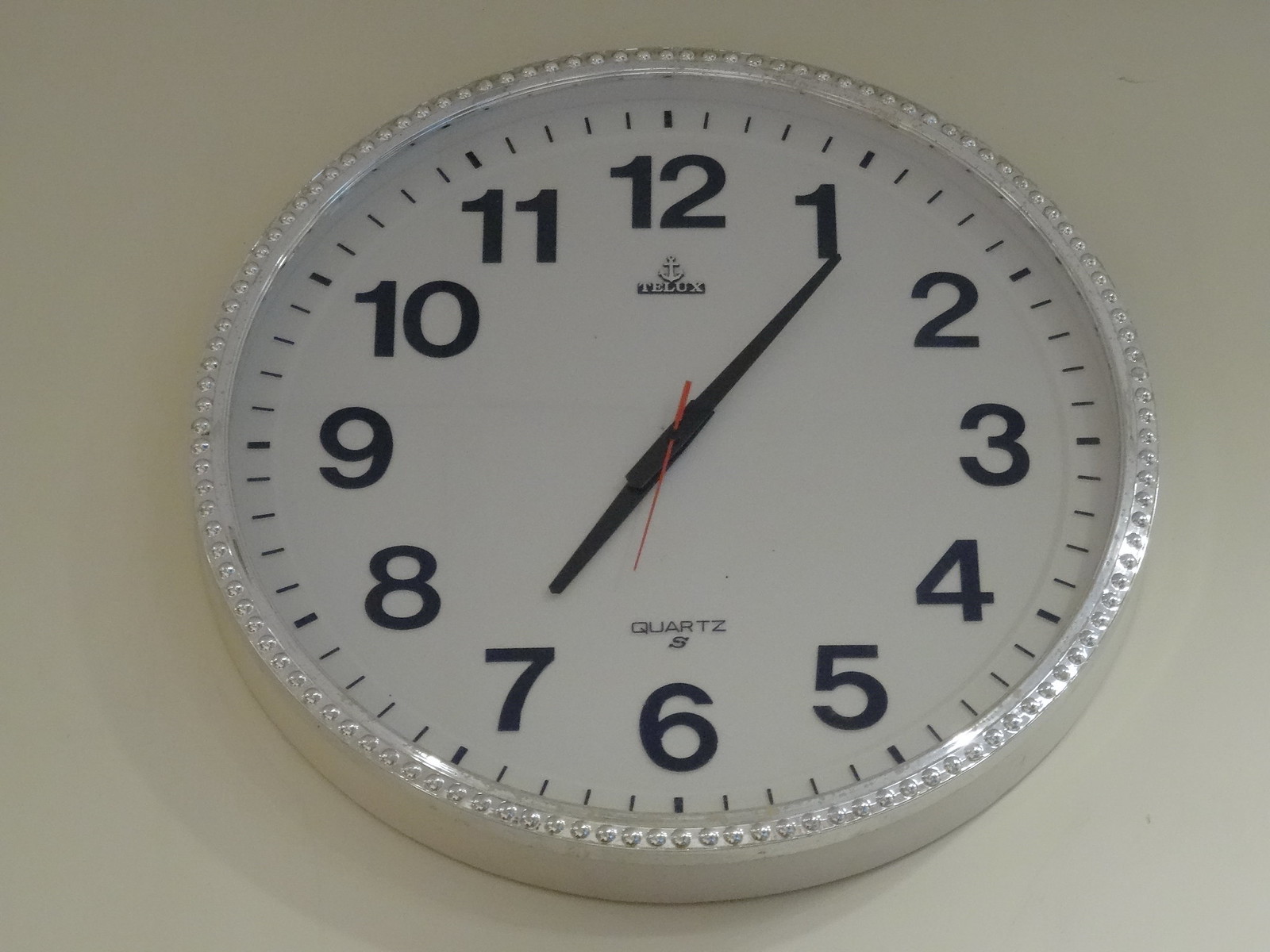This photograph captures a close-up view of a large, round wall clock positioned against a tan-colored wall. The clock, which dominates the entire frame, features a sleek silver exterior bezel adorned with evenly spaced, pearl-shaped dots. The clock's face is classic white, showcasing bold black numerals and standard black hour and minute hands, complemented by a distinct red second hand. Inscribed just above the six o'clock position on the bezel is the word "Quartz," indicating the clock's type. Above the twelve o'clock mark, a maker's mark with a distinctive sailor's anchor emblem gracefully punctuates the design, adding a touch of nautical elegance to the timepiece.